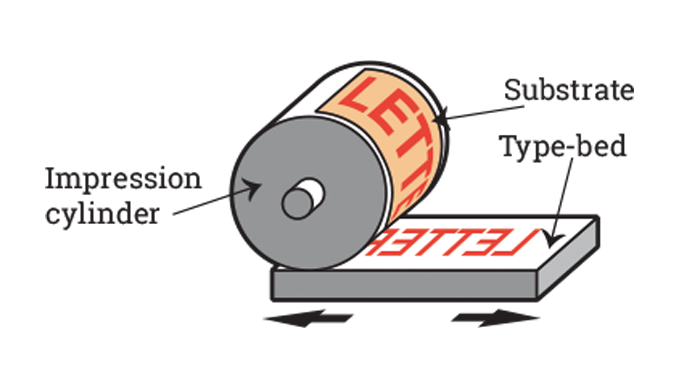This detailed drawing illustrates how a print impression system works. Central to the image is an impression cylinder, labeled accordingly, which features the word "LETTER" in red on a peach-colored background. This cylinder rolls over a rectangular type bed, which has the word "LETTER" imprinted backward, shown on a white surface. The diagram includes various annotations with black arrows pointing to key components: the "impression cylinder" on the left, the "substrate" on the right, which is the inked area on the cylinder, and the "type bed" pointing to the rectangular base that receives the impression. The image uses clip art style to effectively communicate the mechanical process, aiming to teach about the different parts and functions involved in creating a print impression.